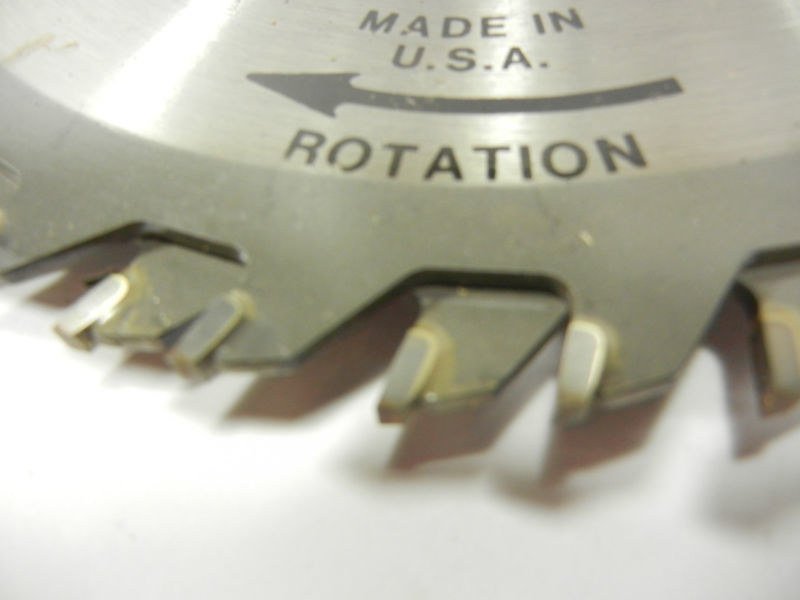This horizontal, somewhat blurry color photograph features a close-up view of a circular cutting blade, resembling those used in sawmills. The edge of the blade appears sharp with visible teeth; specifically, five teeth are clearly discernible in this zoomed-in frame. The blade, made of steel and finished in a silvery hue, rests on a white surface and casts a shadow beneath it. The light from above creates a glare on the metal surface, adding a reflective highlight to the image. Notably, text in black, all-capital letters on the blade reads, "MADE IN U.S.A." and "ROTATION," accompanied by a prominent bold arrow pointing to the left, indicating the correct rotational direction. This photo, likely taken with a personal camera under heavy lighting, captures the detailed textures and markings of the blade.